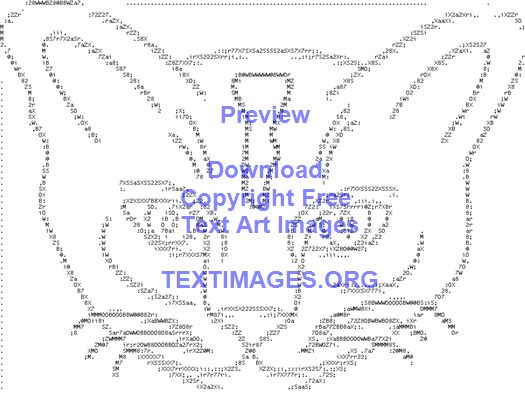The image captures a detailed text art representation of a cat, crafted using numbers, letters, and symbols in a style reminiscent of 1980s computer print on continuous feed paper. The cat’s face, which fills the entire space, features distinct elements like whiskers, eyes, a nose, ears, and a patch in the middle of its forehead. The face is meticulously outlined with numbers and letters, adding to the intricate design. Superimposed over the cat’s face, in large blue text, are the words: "Preview" and "Download", followed by "Copyright Free", "Text Art Images", and at the bottom, "TextImages.org". The paper’s edges are visible on the top and left, but not on the bottom or right, giving the impression of an expansive digital artwork.